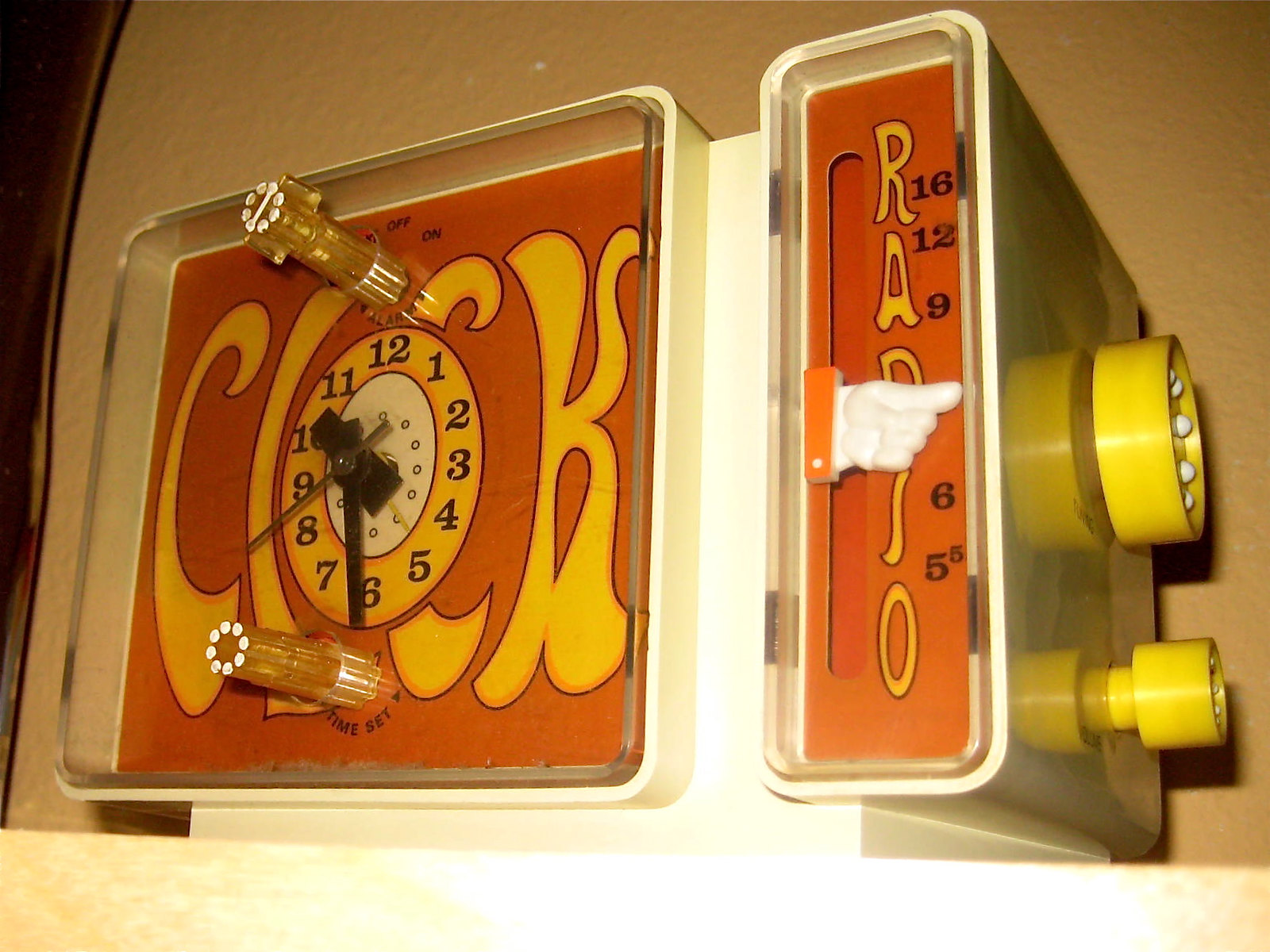This is a photograph of a vintage clock radio, likely from the 1960s or early 1970s, characterized by its distinctive, whimsical font. On the left side of the device, you see a clock with a classic analog face, surrounded by knobs for setting the time. The clock face is cleverly integrated into the typography, with the 'O' in the word "Clock" depicting the clock itself, complete with numerals and clock hands. 

On the right side, the word "Radio" is displayed vertically, with a plastic hand featuring white fingers pointing up and down to indicate the tuning band. Below the word "Radio," the frequencies 16, 12, and 9 are listed, presumably representing AM or FM band markers. The dials used for adjusting these settings are located on the right side of the clock radio. The overall design of the clock radio is nostalgic, with a white and orange color scheme that enhances its retro appeal.